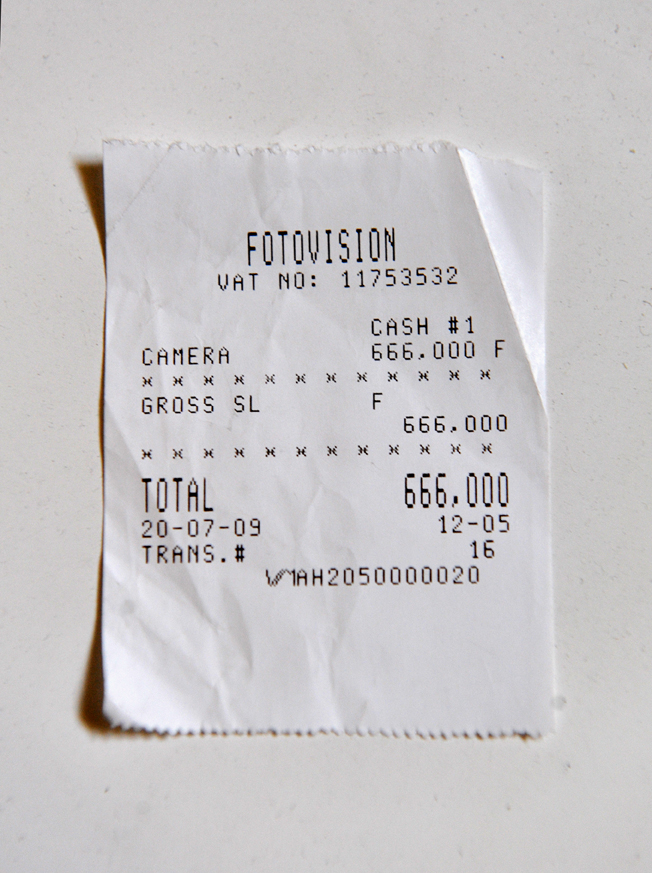The close-up photo showcases a small, white receipt with perforated edges at the top and bottom, indicating it was torn from a machine. The receipt, sitting on a white table, has slightly crimped right edges, perhaps from being folded. At the top, the receipt prominently displays "PhotoVision" in larger, pixelated text. Centered beneath is the VAT number 1175352. Below, it lists the purchase of a "Camera" priced at an astonishing $666,000, denoted with an "F" for the currency. Following a line of X's, the "Gross SL" and "Total" both reflect the same amount of $666,000. The date, formatted as 20-07-09, and time, 12:05, are situated under the total amount, with a transaction number of 16. Further down, an additional reference number "1-AH-20-5-00-00-020" is printed, though its purpose is unclear.